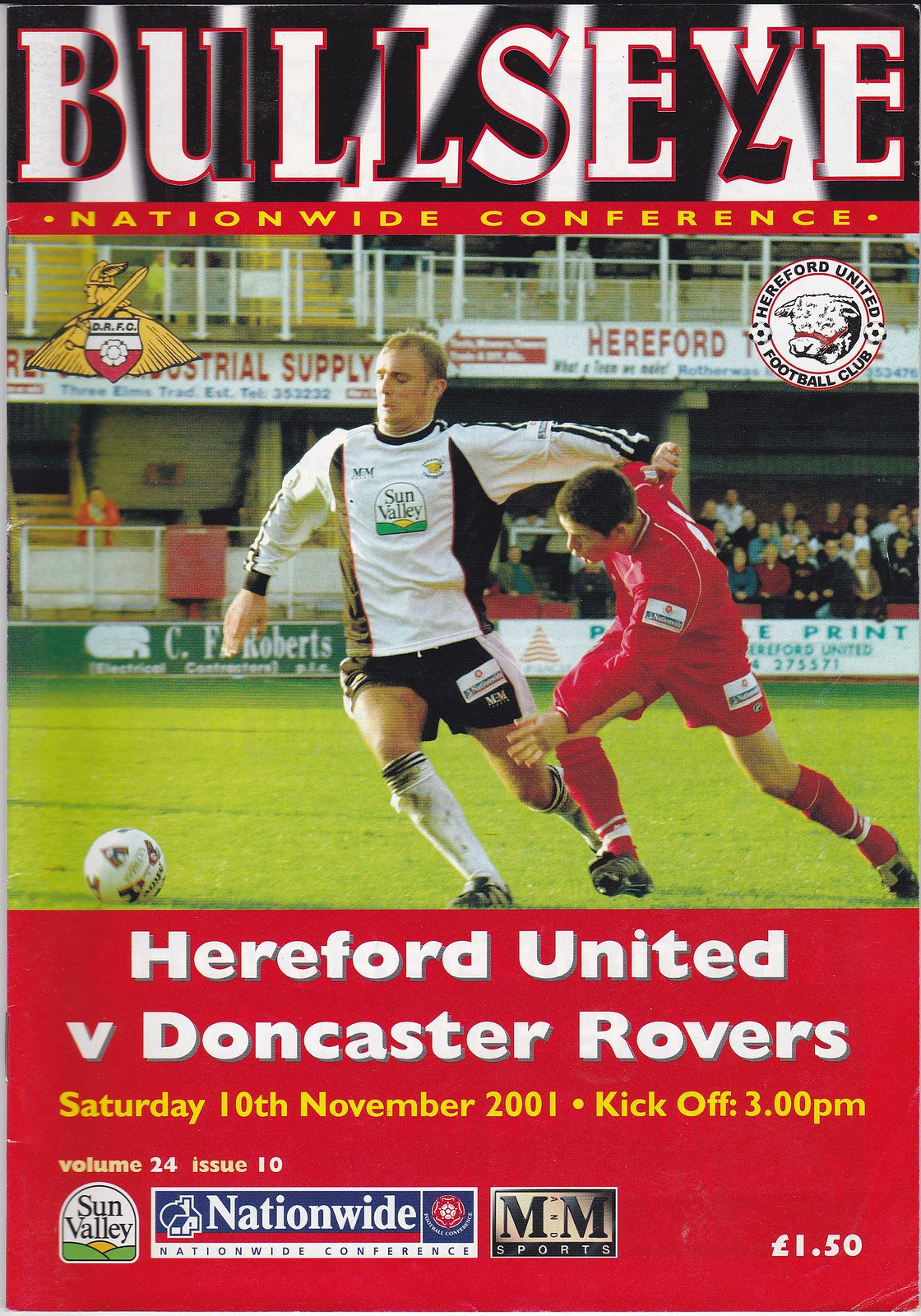The image is an advertisement for a sports game, prominently featuring the title "Bullseye" at the top in large black and white text. Below it, a red stripe spans the width of the image with "Nationwide Conference" written in yellow text. The central focus of the image is a close-up of two men playing soccer on a field, engaged in a vigorous battle for the ball. One man is dressed in a red uniform, including red and white socks, while the other wears a black and white jersey, black shorts, white socks, and black cleats. The background hints at the stadium setting.

Below the players, another red box contains white text that reads, "Hereford United versus Doncaster Rovers," indicating the teams playing. Beneath this box, additional details are provided in small yellow text: "Saturday, 10th November 2001, kick-off at 3 PM." There are also two watermarks: one for "Hereford United Football Club" featuring an image of a cow, and another with the text "DEFC," represented with a gold image of a man with a sword.

Additional branding is present at the bottom of the advertisement, which includes "Sun Valley," "Nationwide," and "MM Sport." The issue details are noted as "Volume 24, Issue 10." Finally, the price is marked as £1.50, indicating the cost in pounds.

In summary, this advertisement effectively combines game information, team insignias, and brand logos to promote the soccer match between Hereford United and Doncaster Rovers.